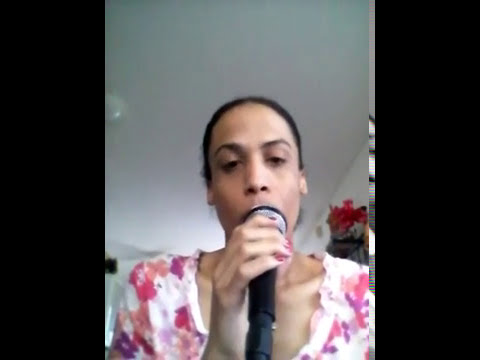The image is a horizontal, rectangular photo bordered on both sides by inch-wide black vertical sidebars. It prominently features a woman singing into a microphone held very close to her mouth, obscuring her lips but leaving her eyes, nose, and ears clearly visible. She is wearing a white dress adorned with pink, red, and purple floral patterns. Her dark hair is pulled back, and both of her hands, which have red painted nails, are visible and free of any obstructions apart from the microphone. The woman appears to be in a room with gray or white walls, possibly a living room or bedroom, and there seem to be flowers on the right side behind her shoulder. Some upper shelving or ceiling space is also faintly visible in the background. The overall image, potentially taken from a lower angle via a cell phone or webcam for a social media selfie, is of medium to low quality, emphasizing a casual, intimate moment.